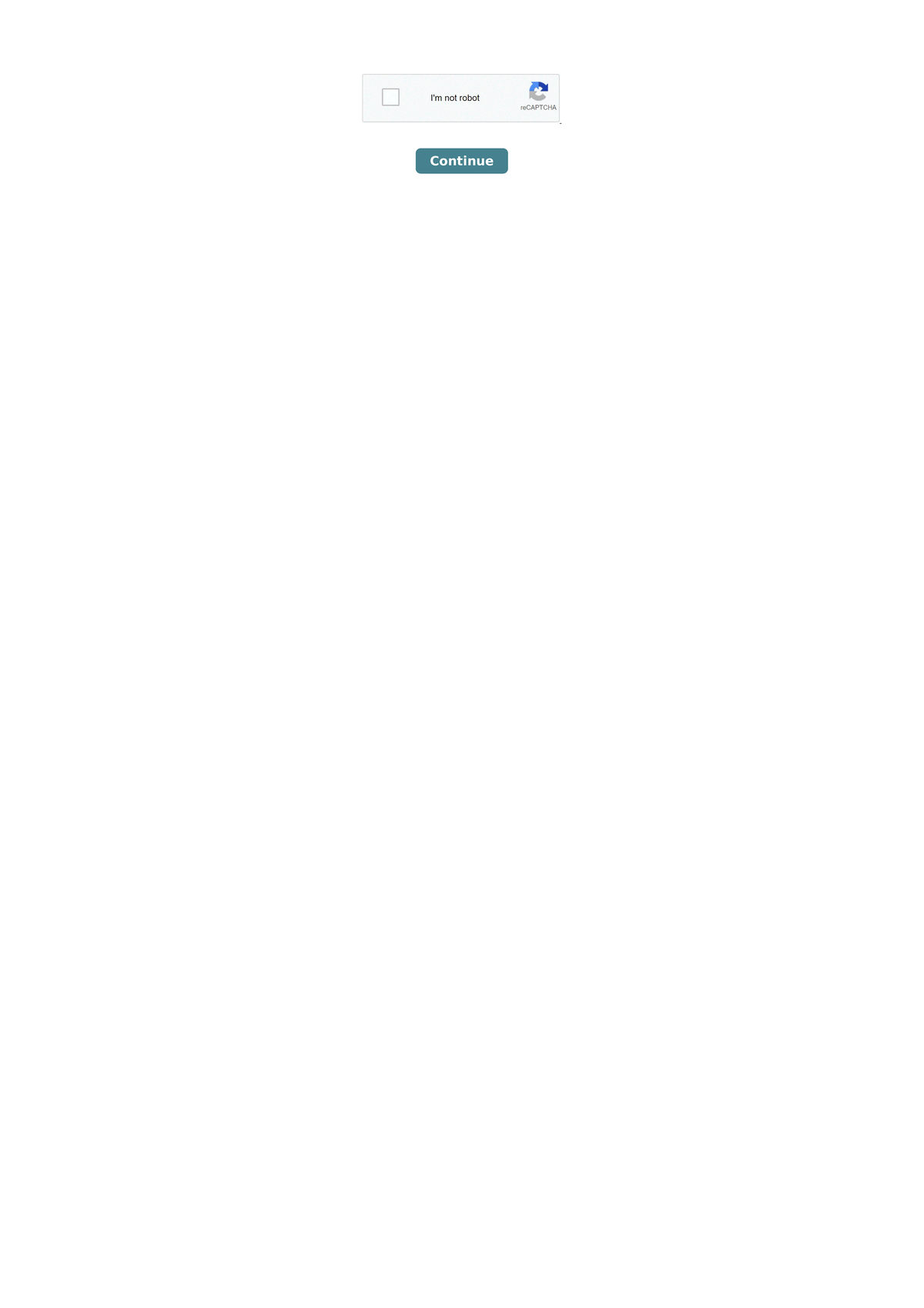The image depicts a minimalistic web page primarily displaying a CAPTCHA verification prompt, designed to distinguish human users from bots. The screen is mostly blank with a white background, except for a centrally located gray rectangle that is roughly three times wider than it is tall. In the left part of the gray rectangle, there is a small white square that users can click to check and verify their humanity. At the center of the rectangle, in a gray font, the text reads "I'm not a robot." On the right side, there is the CAPTCHA logo, which is an open circle with an arrow at its right side. Below this verification area, there is a blue rectangular button featuring white text that says "Continue." The design is clean and straightforward, ensuring the CAPTCHA process is clear and user-friendly.